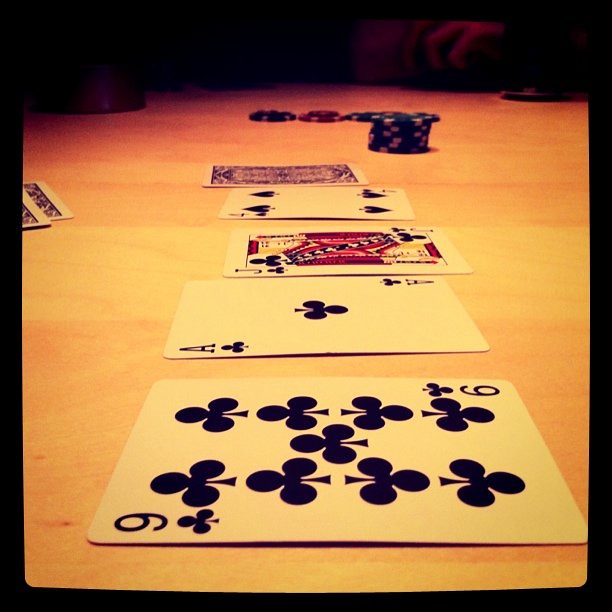The photograph captures an intense moment of a poker game, framed artistically in black. Inside this black frame, the scene is set on a light-colored, gold-shimmering wooden table that serves as the elegant backdrop for the game. Dark shadows of hands engaged in play cast an air of mystery in the upper center of the image, emphasizing the strategic deliberations happening out of sight.

At the lower part of the image, carefully arranged poker chips and cards draw the eye. In the upper center, a neat stack of blue and white poker chips, interspersed with a red chip, signify varying amounts of money, adding to the tension of the game. 

To the left of the center, two cards lie face down, their patterned backs subtly displayed. In front of the poker chips, a similarly patterned card is also face down, propped against a four of spades card. Adjacent to it is a jack of clubs, richly detailed with its royal pattern — flaunting yellow hair, a red and blue crown, and an elaborate red and blue outfit, conveying an air of regality.

Leaning against the jack is an ace of clubs, while front and center lies a nine of clubs. Each of these cards faces from left to right, creating a harmonious composition that draws attention to the flow and arrangement of the game.

The photograph's artistic style and meticulous detail make it a piece worthy of framing and displaying on a wall, perfectly capturing the elegance and allure of a high-stakes poker game.